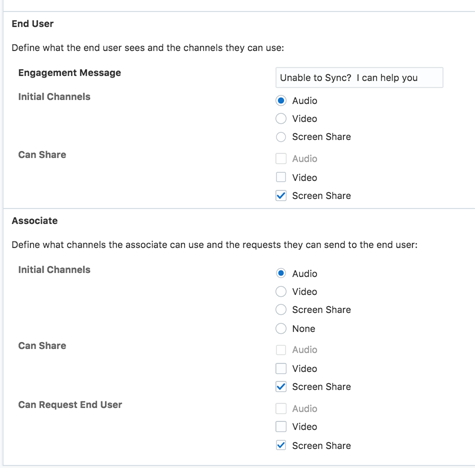This screenshot captures the settings interface of a website or application, presented on a white background with black text. Two outlined rectangles, bordered by faint gray lines, are displayed vertically.

The top rectangle is labeled "End User" in bold black font. Beneath this, it states, "Define what the end user sees and channels they can use:" Following this is a bolded section labeled "Engagement Message," accompanied by a button that reads, "Unable to sync I can help you."

Subsequently, there is a section titled "Initial Channels," offering options for Audio, Video, and Screen Share, with Audio selected. Following this is a section titled "Can Share," presenting the same options—Audio, Video, and Screen Share—with Screen Share selected this time.

The second rectangle, labeled "Associate," directs, "Define what channels the associate can use and requests that they can send to the end user:" It provides options for "Initial Challenge Channels," which include Audio, Video, Screen Share, and None, with Audio selected. Another section, "Can Share," offers the same options—Audio, Video, and Screen Share—with Screen Share selected.